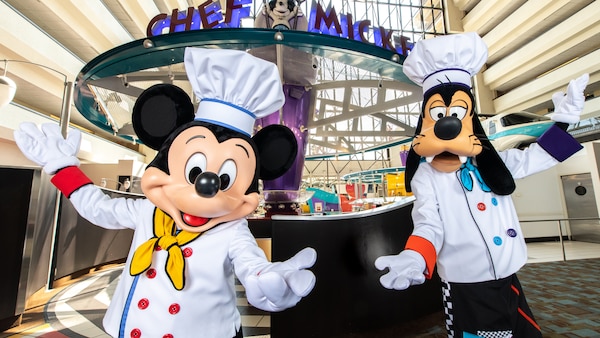In the image, a vibrant scene is set in a Disney-themed hotel or food court, with a clear sign above the buffet area reading "Chef Mickey." Front and center, Mickey Mouse and Goofy enthusiastically present themselves in full chef attire. Both characters don white chef's coats and hats. Mickey's outfit is detailed with distinctive red buttons, a bold yellow tie, and a red cuff on his right arm, while Goofy's outfit showcases a mix of blue, red, and purple buttons, a blue tie, and cuffs that are uniquely colored—orange on one arm and navy blue on the other. They are both wearing black pants accented with white checkers on the sides. Mickey and Goofy, with their signature smiles and Goofy's prominent buck teeth, have their arms spread wide as if presenting something grand, adding to the cheerful and welcoming atmosphere. The attention to the vibrant and differing details of their attire highlights the playful and meticulous theming typical of Disney environments.